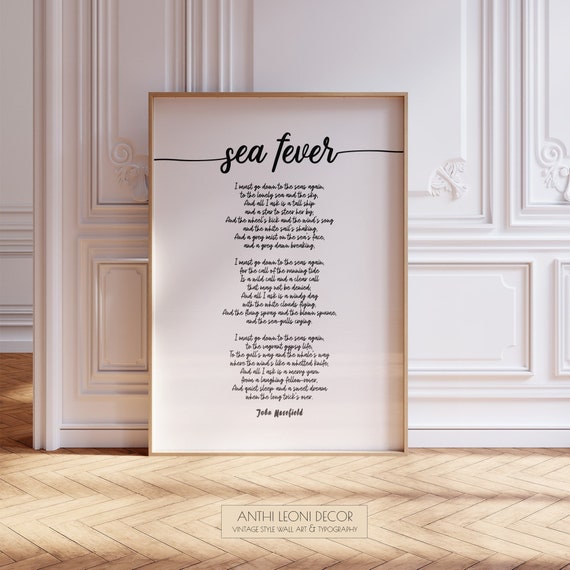The image features a large framed piece of artwork titled "Sea Fever," leaning against an ornate white wall characterized by intricate molding and framed panels. The floor beneath is made of light blonde wood, arranged in a chevron pattern of diagonal and horizontal slats. The poem "Sea Fever" is written in a cursive font, beginning with the line "I must go down to the sea again to the lovely sea and sky and all I ask is a tall ship and a star to steer her by." The text is set against a white background and enclosed in a thin, goldish wooden frame. At the very bottom of the image, a small brown label reads "Anthe Leoni Decor Vintage Style Wall Art and Typography," adding a touch of vintage elegance to the overall decor.